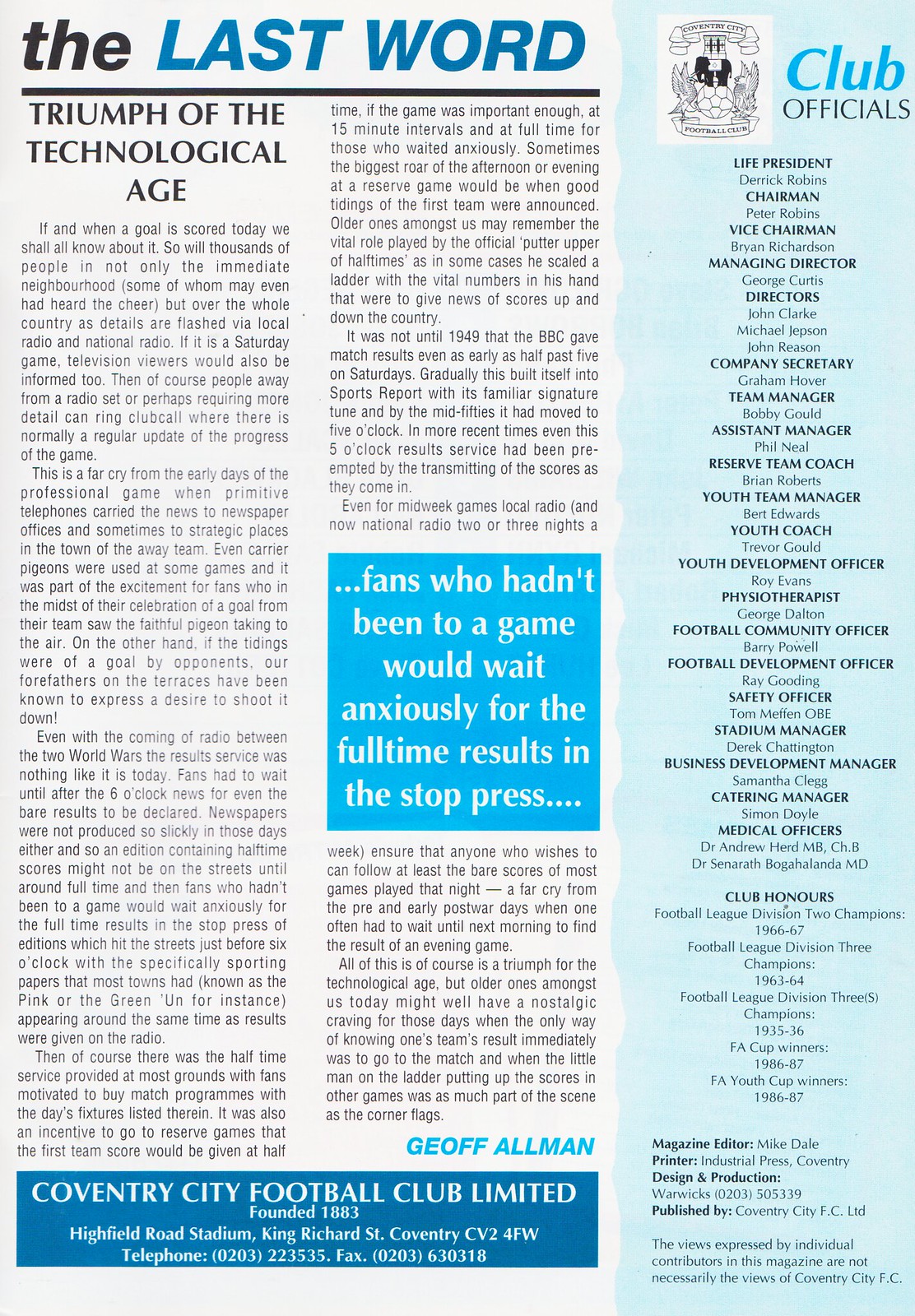This tall rectangular image appears to be a scan of a magazine page or a poster comprising three columns. The left and middle columns are set against an off-white background, while the right column has a very light blue background, separated from the rest by a squiggly line. At the top of the left white column, bold lettering spells out "the last word," with "the" in black font and "last word" in blue. Just below this, the title "Triumph of the Technological Age" introduces a two-column article. Midway through the article, a bright blue square with white text highlights the quote, "Fans who hadn't been to a game would anxiously wait for the full-time results in the stop press." 

The content includes about six paragraphs elaborating on the topic, authored by Jeff Bauman. Beneath this article, there is a blue and white advertisement. The right column details a list of individuals associated with a football club, labeled "convention city football club limited" and founded in 1883. It includes their Highfield Road Stadium address at King Richard Street, Century CV2 4FW. The column lists various club officials such as the president, chairman, vice chairman, managing director, youth development officer, youth team manager, club honors business development manager, and football community officer.